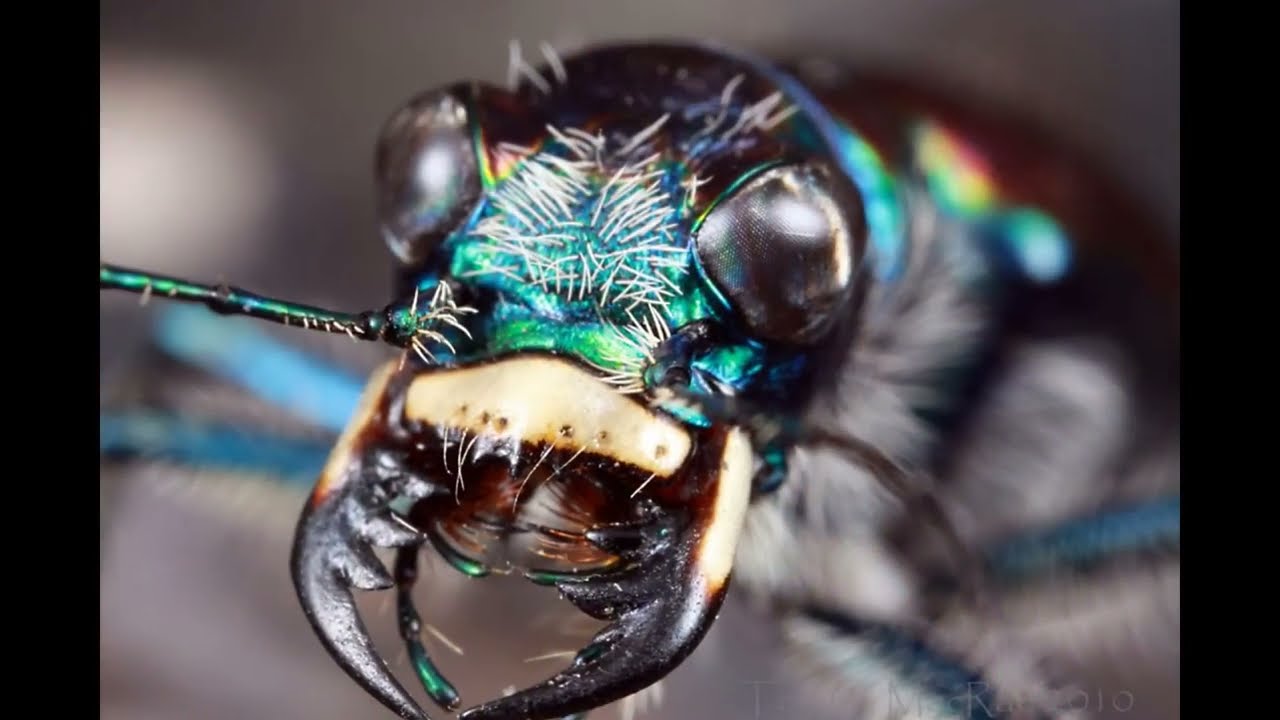The image presents a hyper-close-up, macro photograph of an insect, predominantly focusing on its head. This insect resembles a fly but appears even more intricate and menacing. The head, vividly iridescent with hues shifting between purple, blue, green, and hints of yellow and red, is sharply in focus against a blurred, indistinct background. The insect's body fades out of clarity, with only a glimmer of its long, shining legs visible, reflecting a bluish metallic sheen.

Dominating the insect's face are two large, black, bulging eyes that seem to stare directly at the viewer. Between these eyes, clusters of fine, white hairs jut out, contributing to the insect's intimidating appearance. The top of the head is covered in black, hairy texture.

The insect's mouth is notably fearsome, equipped with projectile-like appendages extending from its purple, blue, and green center. These pincers or claws are dark and formidable, positioned to capture and drag prey towards the insect's mouth. They feature sharp points and segmented, fang-like structures along their inner edges, with a bone-white coloration near their base, adding to the overall threatening aspect of the insect. The entire composition, framed by black bars on both sides from top to bottom, enhances the intensity and focus on the insect’s otherworldly visage.